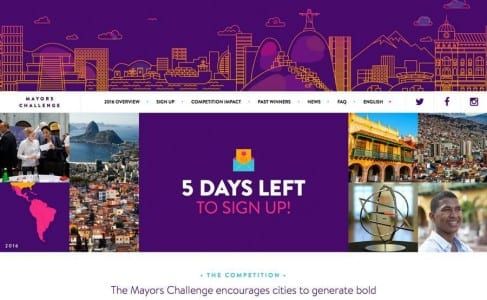This screenshot showcases a visually striking webpage with a prominent purple theme. At the top, a captivating background image features an artistic outline of a cityscape against purple hills and mountains. The outlines of the buildings and the landscape are highlighted in gold, adding a touch of elegance to the scene. Below this graphic, a white navigation bar spans across the middle of the page. On the left side of the bar, text mentioning "challenges" or "challenge me" is partially visible. To the right, there are seven text buttons labeled as "Overview," "Sign Up," "Competition," "Impact," "News," and "FAQ," with the language set to English.